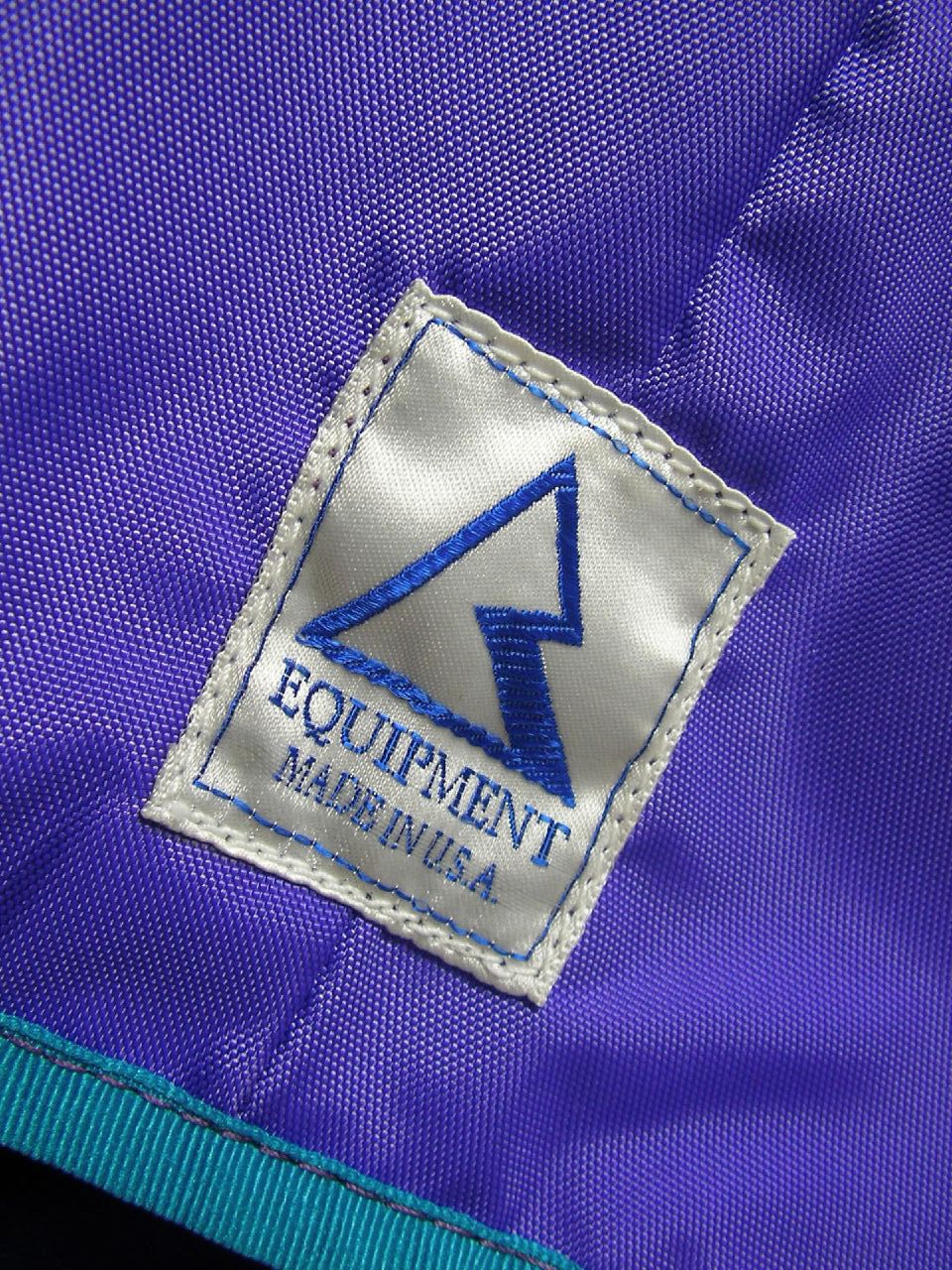The image depicts a blue item, made from polyester material. It appears to be either a bag or a cover. The fabric is a rich, royal blue color, accented with an aqua-colored border along the edge. Inside, there is a white patch with the text "Equipment Made in USA" sewn onto it. The patch is bordered with white stitching, while an additional line of blue stitching forms an inner border. The patch features a unique logo: a triangle that transforms into an arrow, pointing downward.